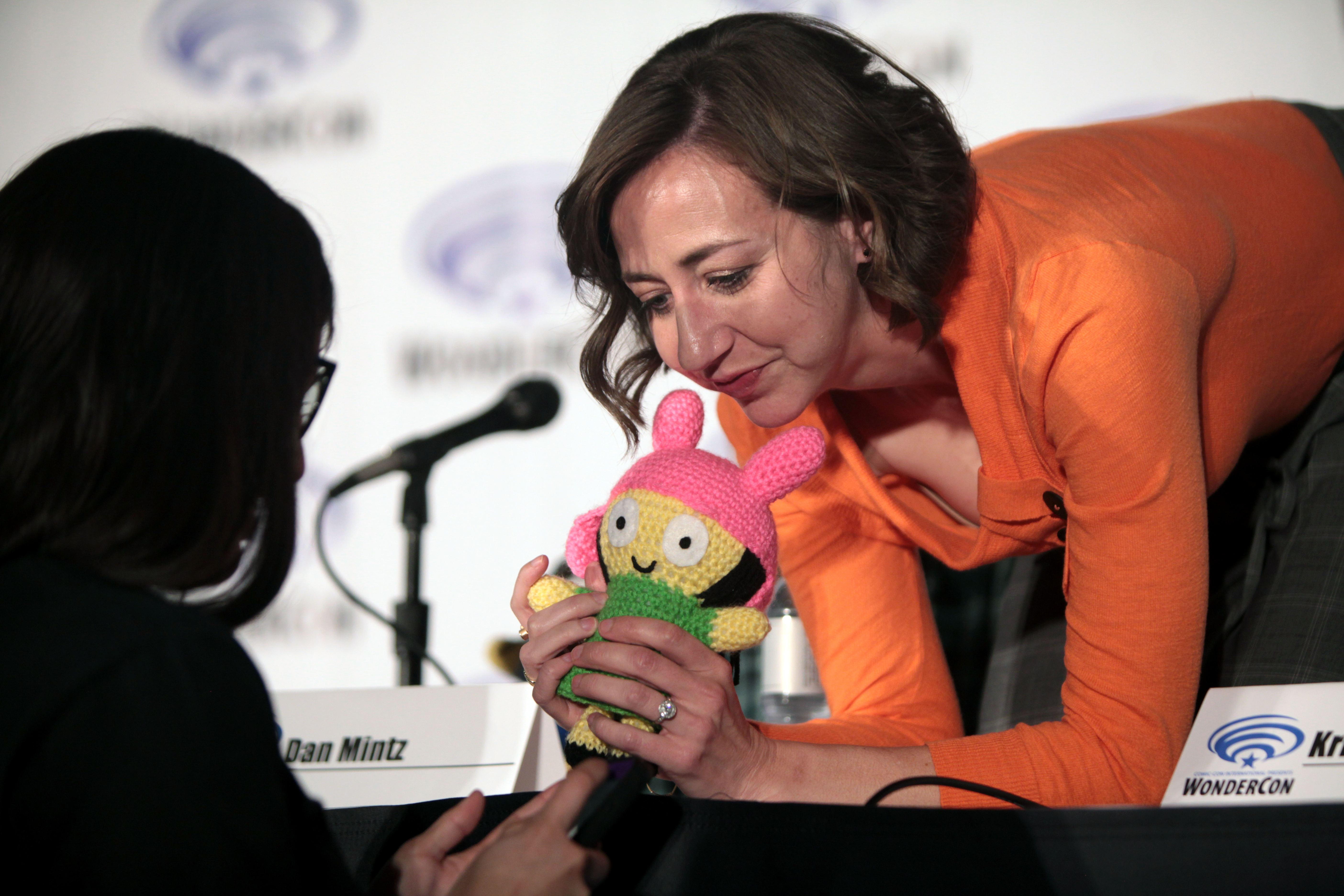In this photograph, a woman in an orange long-sleeve shirt and gray pants is leaning over a table adorned with a black tablecloth and name tags. She is warmly accepting a crocheted plush cartoon character, which wears a green skirt and a pink bunny hat, from a person partially visible in the photo’s bottom left corner. The person has black hair, wears glasses, and is seen wearing a dark-colored shirt. The plush character is gently held in the woman's hands, displaying her wedding ring. The table is partially covered with white name tags, including one that reads "Dan Mintz" while another is mostly cut off, showing only a "K." The setting appears to be a conference room, reinforced by a backdrop with symbols and wording and a microphone visible on the table, though the details of the backdrop are blurry and unidentifiable. The woman’s posture and the surrounding elements—colors of orange, pink, green, and black—suggest a moment of heartfelt interaction, likely captured indoors during an event.